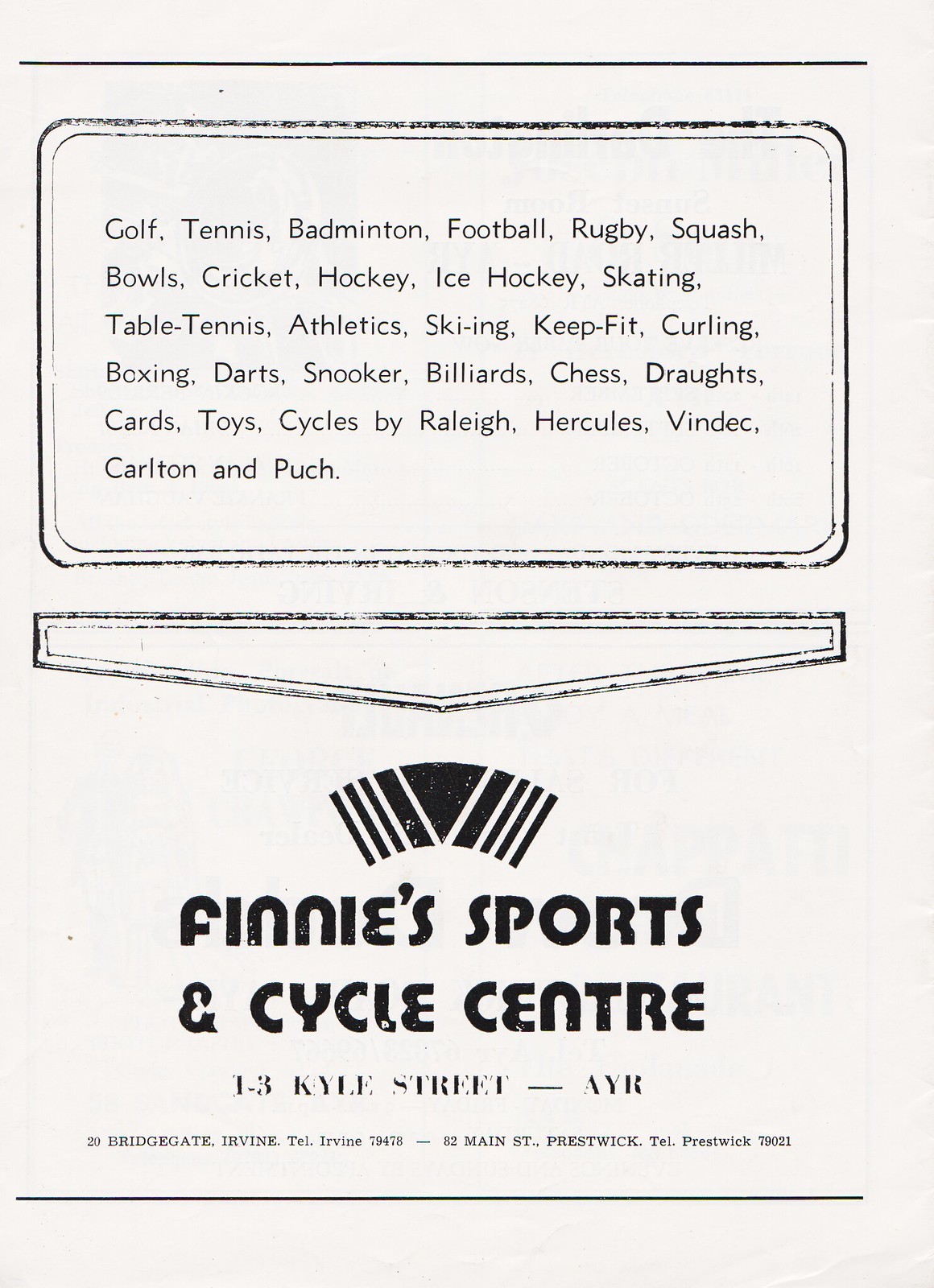This black-and-white image depicts a slightly creased paper flyer advertising Finney's Sports and Cycle Center. The top section features a large list of products and activities available, written in black text. These include: golf, tennis, badminton, football, rugby, squash, bowls, cricket, hockey, ice hockey, skating, table tennis, athletics, skiing, keep fit, curling, boxing, darts, snooker, billiards, chess, draughts, cards, toys, and cycles by Raleigh, Hercules, Vindec, Carlton, and Puch. The bottom section of the flyer displays the Finney's Sports and Cycle Center logo, with bold black text and an arch-shaped decoration. The addresses listed are 1 to 3 Kyle Street, Ayr; 20 Bridgegate, Irvine; and Main Street, Prestwick, along with their respective telephone numbers Irvine 794-78-82 and Prestwick 790-21.